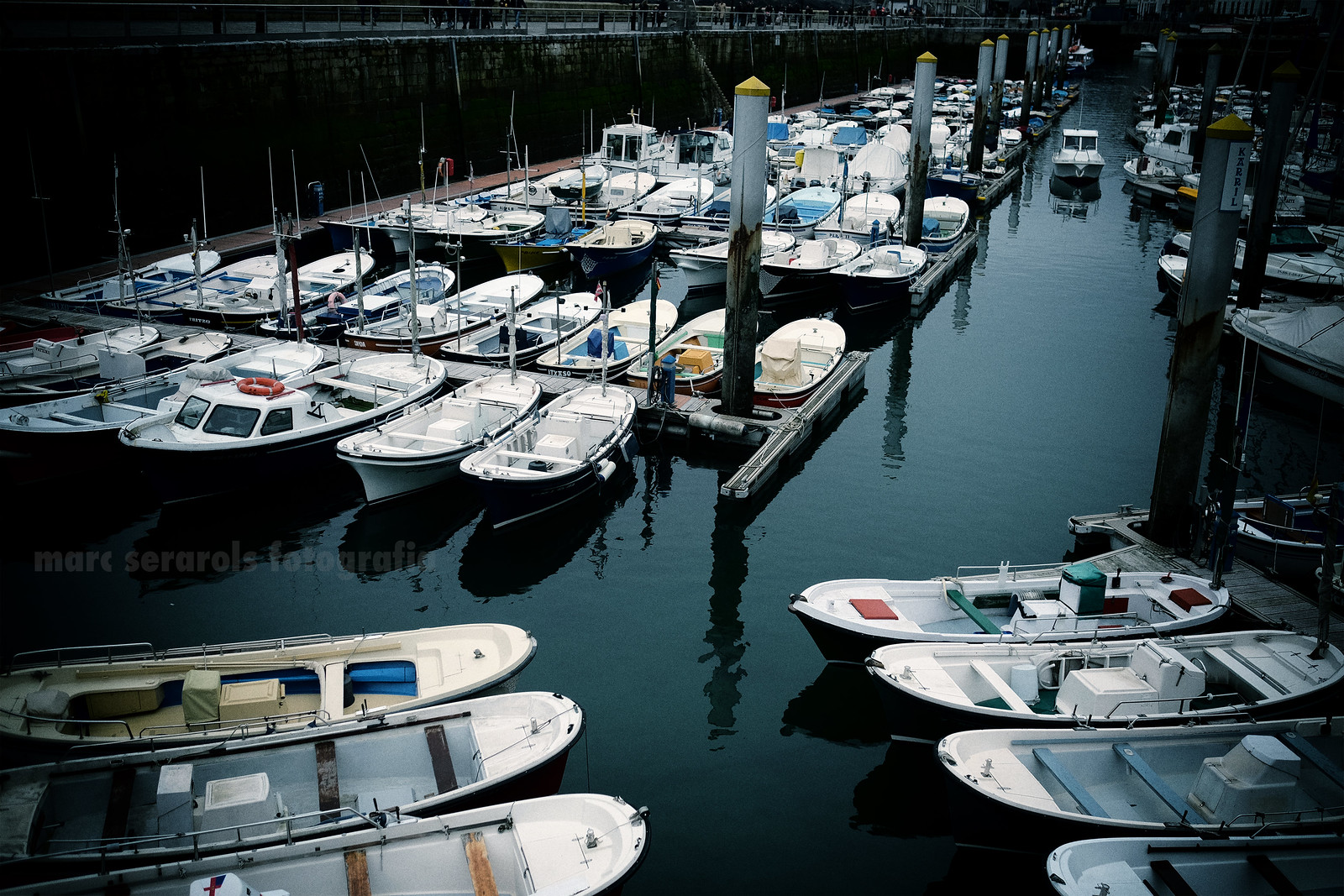This is a detailed photograph of a bustling marina, captured with a distinct watermark reading "Marc Serralo Photography." The scene features six rows of piers extending into the water, each lined with more than a dozen boats. These boats vary in design, with some being small speedboats and others equipped with cabins or containers. The boats are neatly arranged side by side, creating a pattern of diagonal and straight lines across the harbor. The piers are interconnected by walkways, with posts lined along the water. At the lower corners of the image, there are boats with blue wooden boardings and others with white finishes, some featuring seating areas. Notably, one boat is seen navigating through the waterway, adding a dynamic element to the dense and orderly arrangement. The overall image is presented with a dark, dense filter, enhancing the contrast and details of the marina scene.